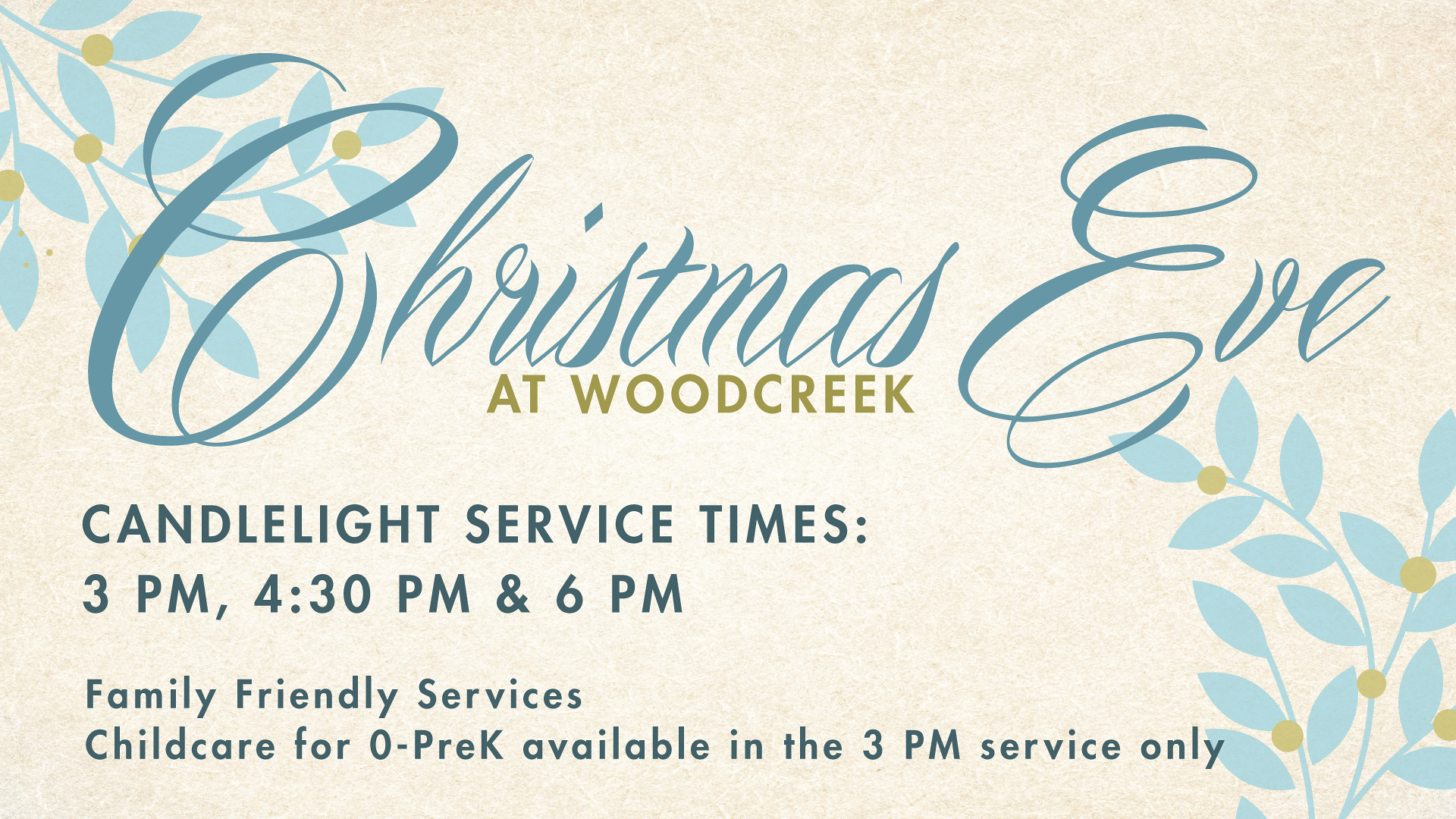This image is an advertisement for a Christmas Eve church service, featuring a subtle tan paper background with blue floral designs in the upper left and bottom right corners. The centerpiece of the design prominently displays the text "Christmas Eve" in elegant blue cursive, with "at Wood Creek" written in gold beneath it. Below, in darker blue, are the Candlelight Service times: 3 p.m., 4:30 p.m., and 6 p.m. Additional information highlights that these are family-friendly services, with childcare for children from zero to pre-k available only during the 3 p.m. service. The overall aesthetic is festive yet understated, offering a welcoming invitation to both the community and regular churchgoers.